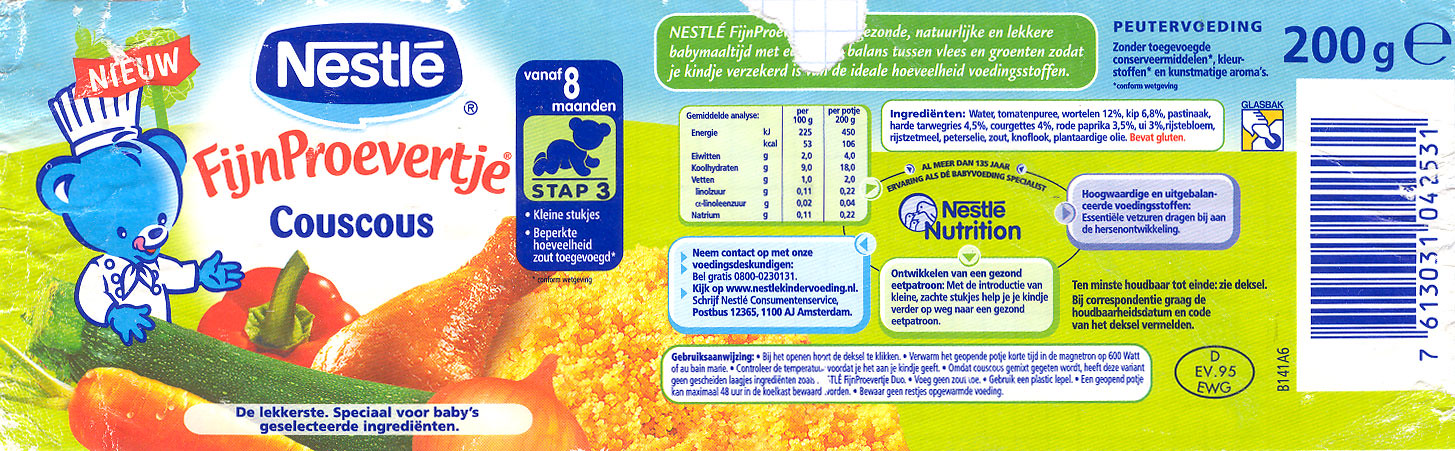This vibrant and colorful label belongs to a Nestlé baby food product. A delightful medley of imagery showcases fresh ingredients, including red bell pepper, zucchini, carrots, onions, chicken, and rice, against a lively blue background. The label also includes essential information such as nutrition facts, a UPC code, and the product weight. Despite being in a language different from English, the label prominently features a picture of a baby, indicating that it is indeed intended for infants. A bold statement declares it as a new product, adding to its appeal.